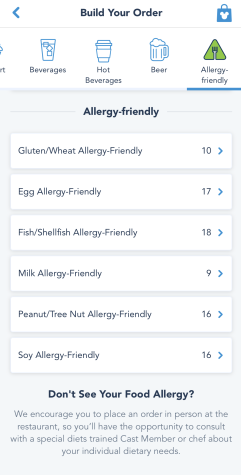In this screenshot of the Disney app, likely for Disneyland or Disney World, the top section displays "Build Your Order" in bold text. To the right of this text is a blue shopping bag icon featuring a white Mickey Mouse symbol, and to the left, there's a blue arrow indicating a return to the previous page. Below this, there are segmented tabs for various categories of food and beverages: Beverages, Hot Beverages, Beer, and Allergy-Friendly options, each identified with a distinct icon.

The focus is on the Allergy-Friendly category, which presents multiple sub-categories including: Gluten/Wheat Allergy-Friendly, Egg Allergy-Friendly, Fish/Shellfish Allergy-Friendly, Milk Allergy-Friendly, Peanut/Tree Nut Allergy-Friendly, and Soy Allergy-Friendly. Each sub-category has a number on its right side, likely indicating the number of items available. At the bottom of the screen, a disclaimer in fine print advises customers with food allergies that if their specific allergy is not listed, they should place their order in person at the restaurant to consult with a cast member or chef specializing in special diets. This ensures their individual dietary needs are met. The screen is primarily informative, providing options to accommodate various dietary restrictions.